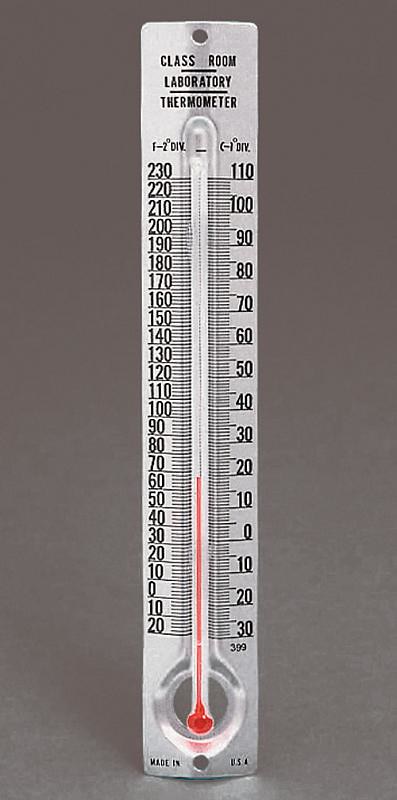The image features a classroom laboratory thermometer, predominantly crafted from silver metal. The top of the thermometer features a hole, suggesting it can be hung for convenience. Inscribed at the top are the words "Classroom Laboratory Thermometer."

The thermometer displays temperature readings on both sides, with Fahrenheit on the left and Celsius on the right. The Fahrenheit scale ranges from 30°F to 230°F, while the Celsius scale ranges from -20°C to 110°C. 

In the center of the thermometer, encased within a glass or plastic tube, is a white rectangular strip marked with black text and multiple dash marks. A red substance, likely mercury or perhaps a red-colored alcohol, is currently at the 20°C (68°F) mark, with the Fahrenheit reading close to 70°F. 

At the bottom of the thermometer, the fine print reveals it was made in the USA. The overall craftsmanship exudes a utilitarian yet robust design, characteristic of scientific instruments used in educational settings.